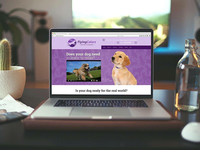A cozy home office setup features a small silver laptop, elevated on a brownish-red ergonomic pad designed to improve typing comfort. The laptop's screen displays a pet-related website with a vibrant purple background, showcasing an adorable golden retriever puppy with a shiny yellow coat and a curious black nose. An embedded YouTube video is also visible on the site next to the puppy. To the left of the laptop, there is a white ceramic cup holding a small green cactus, its shape humorously resembling a pickle. On the right side of the desk, a glass bottle of water sits within easy reach. In the background, a large window or possibly a television screen displays a serene landscape view, adding a touch of tranquility to the workspace.